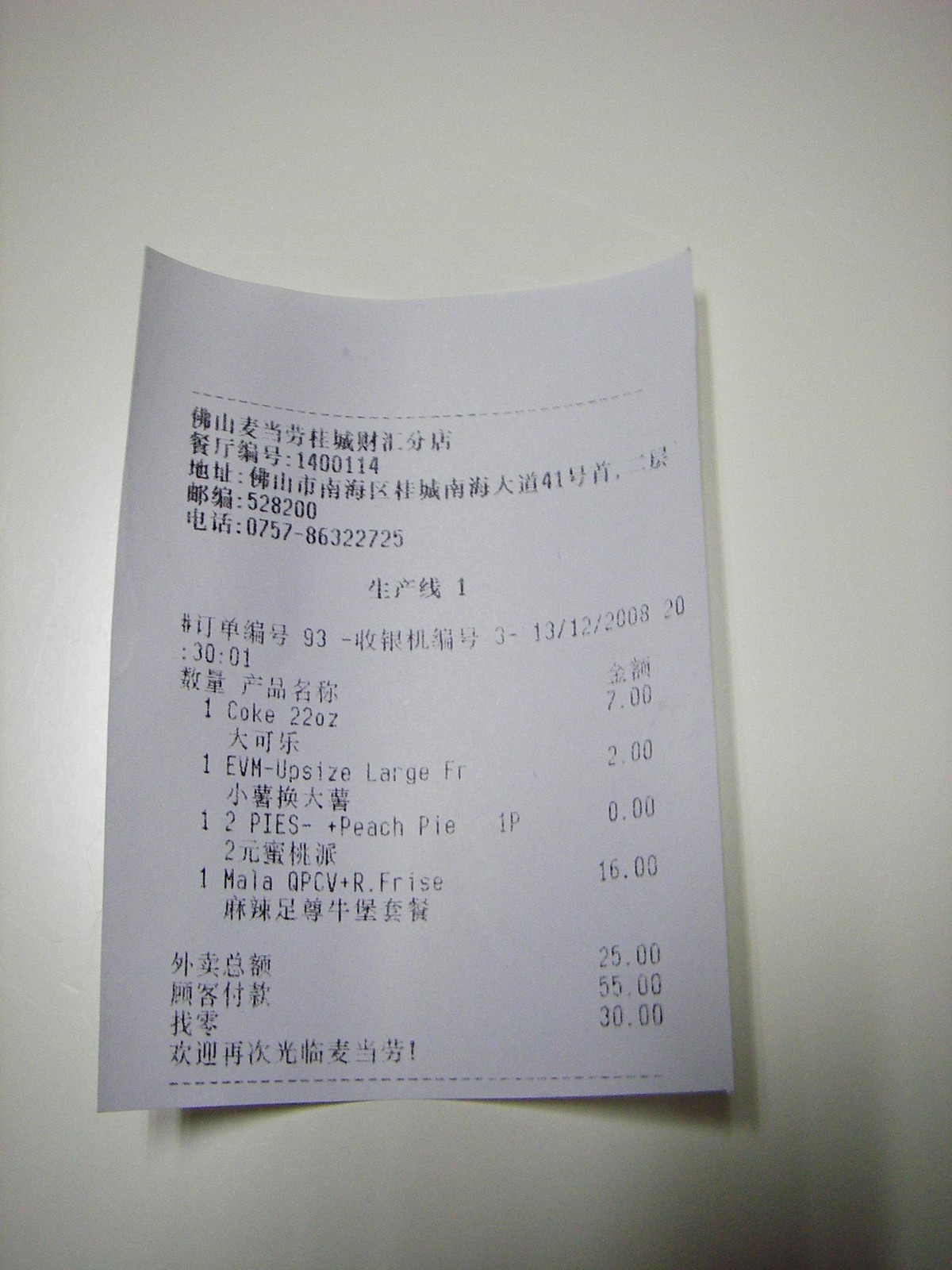This photograph captures an old-fashioned register receipt printed on traditional register paper, placed against a light gray surface. The text on the receipt is in either Chinese or Japanese, making it difficult to comprehend for someone not familiar with these languages. Additionally, the print is very small, limiting legibility. The grand total is $55, as observed on the right side of the receipt. The bill lists five items, culminating in this total amount. The image offers a nostalgic glimpse into retail transactions, characterized by the tactile and visual qualities of paper receipts.